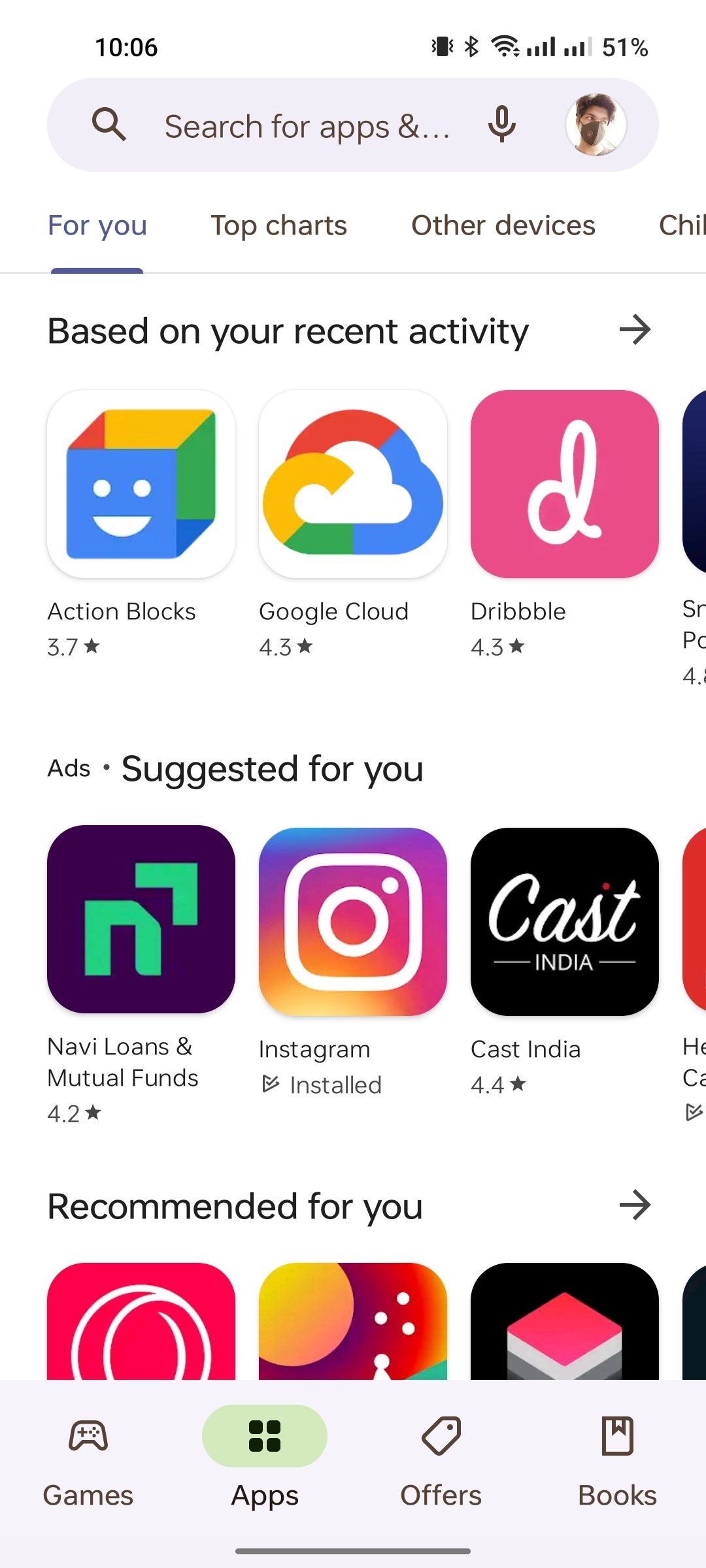A detailed screenshot of an app store interface displays a toolbar at the top featuring the time "10:06" and a battery level indicator at 51%. A search bar is positioned below with a magnifying glass icon indicating the search function, and a microphone icon for voice search. Below the search bar is a profile picture, followed by various sections including "For You," "Top Charts," and "Other Devices Based on Your Recent Activity," with a right-facing arrow for navigation.

The "Apps" section includes listings such as "Action Blocks" with a rating of 3.7, "Google Cloud" rated 4.3, and "Dribbble" with a 4.3 rating. Additionally, there are ads labeled "Suggested for You," featuring "Navi Loans and Mutual Funds" with a 4.2 rating. The "Instagram" app is shown as installed, while "Cast India" boasts a 4.4 rating. Several apps are partially cut off under the "Recommended for You" category.

The background of the interface is white. At the bottom of the screen, there are four navigation icons, for "Games," "Apps" (highlighted with a green circle indicating it is selected), "Offers," and "Books."